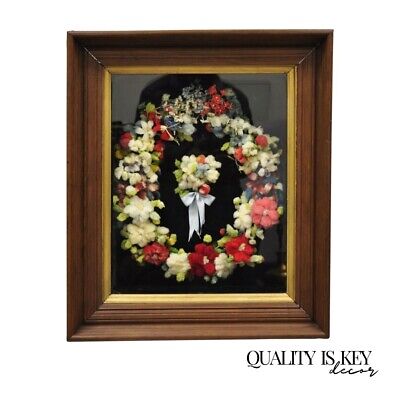The image showcases a detailed and ornate picture frame with a multi-tiered border. The outermost border is a thick brown color, followed by thinner brown layers, and an innermost goldish border. Encased within this frame is a black silhouette of a person, partially obscured by a prominent wreath of flowers. This wreath contains an array of pink, red, and beige flowers, as well as some green puffy blossoms. At the center of the wreath is a smaller bouquet, reminiscent of a bridal arrangement, tied with a light-colored bow. The frame rests against a white background. In the lower right-hand corner of the image, the text "QUALITY IS KEY" is inscribed in bold black lettering, with a cursive word, likely "decor," underneath it. The floral arrangement and intricate details enhance the elegance of the silhouette, making for a unique and captivating composition.